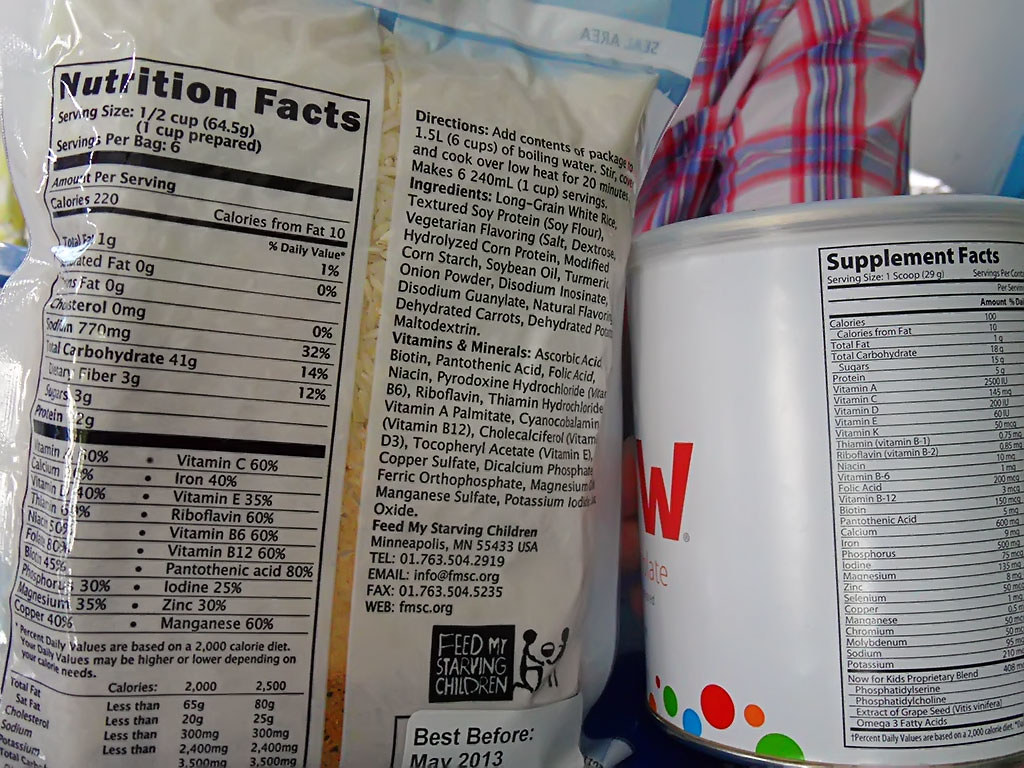In this slightly horizontally rectangular image, we are presented with the back views of two different product packages. Dominating the left side of the frame is a clear bag with a white background, prominently displaying a nutrition facts box. Alongside the nutrition information, there is a transparent vertical window through which we can see what appears to be rice inside the packaging. The other half of the bag contains the directions and ingredients list. Adjacent to this bag and occupying the right side of the image is a round, cardboard-type container with a plastic lid. This container also has a white background and is positioned to show the left-hand side of the supplement facts box, with the right side extending beyond the edge of the frame.